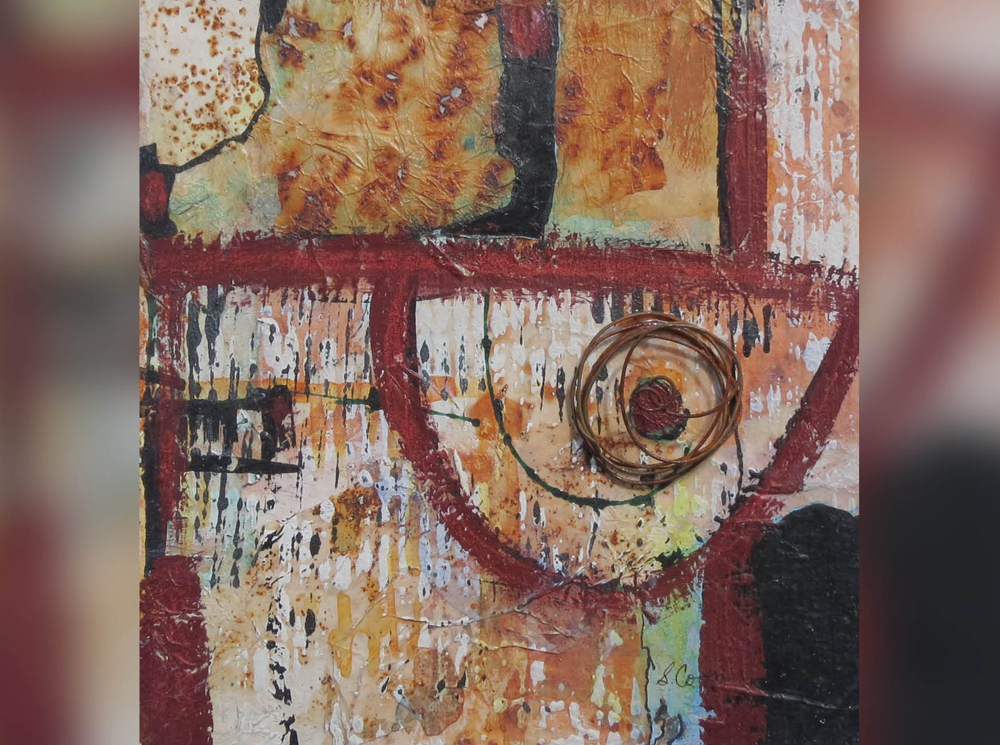This abstract, multi-medium artwork features a central piece that seems to be painted on a piece of wood, set against a backdrop that mirrors and blurs the same image to create depth. The painting is a vivid and textured composition of various colors, prominently showcasing dark maroon red, orange, black, white, peach, gray, turquoise, light blue, and light green. A distinct element is a maroon red border that runs throughout different sections of the painting, emphasizing its abstract form.

In the middle of the artwork is a striking feature: a loop made of an indeterminate material, possibly leather or metal, spirals outward from a central maroon dot, creating a layered and dynamic focal point that resembles an eye. This loop is surrounded by a complex interplay of colors including beige, peach, and orange, adding to the piece's rich textural feel.

There are also notable streaks and splotches of color throughout the painting. A vertical white streak runs up and down the image, and there's a black splotch on the right side, adjacent to a similarly sized maroon section. Rust or burnt-like textures blend into the background, adding to the layered and painterly effect. In addition, sky blue and chartreuse green spots add pops of brightness amid the predominantly warm color palette.

The blurred background painted in similar hues further accentuates the central piece, offering an impressionistic echo of the primary artwork. Subtle textures and a signature, possibly reading "S-C-O-N", can be seen faintly amongst the layers of paint, lending an additional layer of intrigue and complexity to the piece.